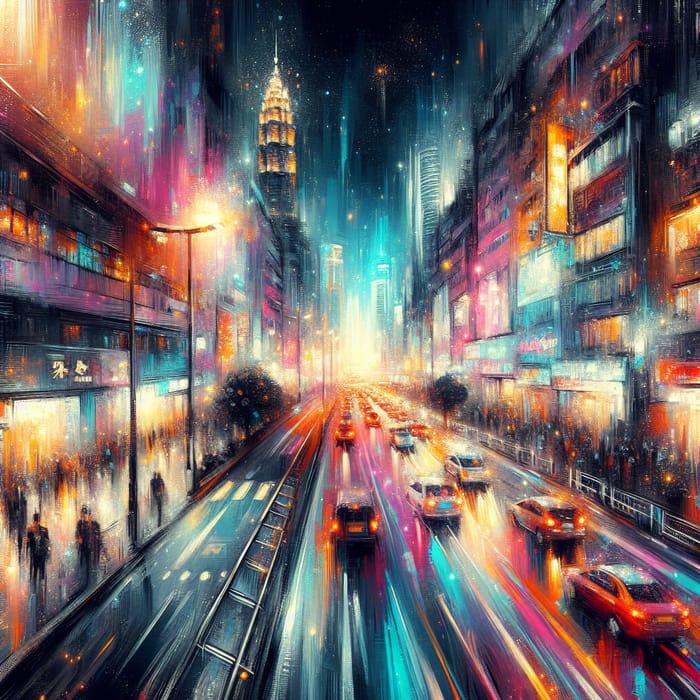The image captures a vibrant, nighttime cityscape that resembles an impressionistic painting. The scene is filled with skyscrapers on both sides of a bustling street, their structures blurred into striking smears of light and color, evocative of a time-lapse photograph or a rain-soaked lens. On both the left and right sidewalks, indistinct figures of people are visible, navigating their evening amidst lampposts and blurred outlines of buildings. The street itself is a riot of pastel hues—purples, blues, aquas, whites, oranges, yellows, and pinks—though notably absent is green. Traffic flows away from the viewer, forming a line of cars also rendered indistinctly, their forms merging into the kaleidoscopic scene. Dots in the sky hint at stars, blending into the ethereal mosaic of the city night. In the background, towering structures fade into the dark expanse above, cementing the picture's dreamlike, almost surreal ambiance. The overall vertical composition of the image further accentuates the grandeur of the city, every element softly blurred into an intricate dance of colors and lights.